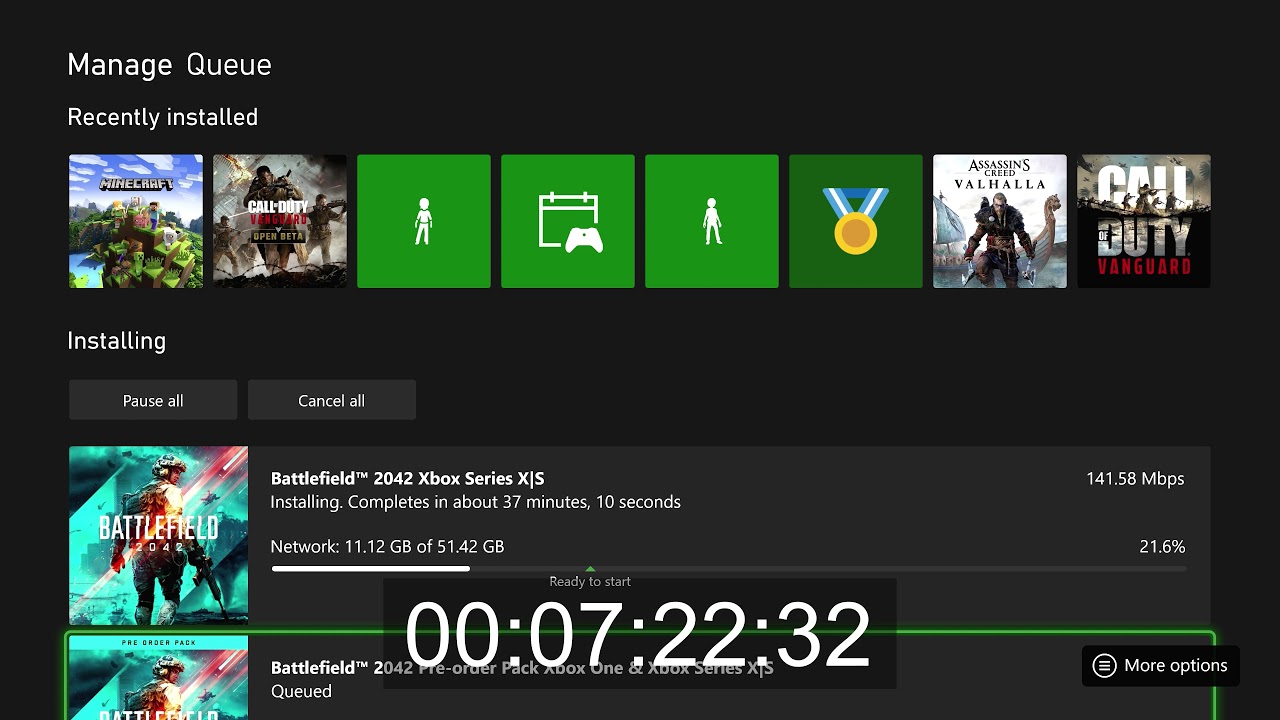The image captures the screen of an Xbox device during the process of managing game downloads and installations. The background is predominantly black, with the top left corner displaying "Manage Queue" in white font. Below it, there is a section labeled "Recently Installed," featuring the cover art of eight different games. The games displayed from left to right are:

1. Minecraft
2. Call of Duty
3. A solid green box with a white stick figure dressed in a shirt and pants.
4. Another green box featuring a white calendar icon and an Xbox controller.
5. A second similar green box with a white stick figure standing with legs positioned differently.
6. A dark green icon showcasing a blue ribbon medal with a gold center.
7. Assassin's Creed Valhalla
8. Call of Duty Vanguard

Beneath these icons, on the left, there's text reading "Installing," followed by two grey buttons with white lettering: "Pause All" and "Cancel All." Below this, the current downloads are listed. 

The first download is "Battlefield 2042 Xbox Series XS." To the left of this entry, the game's cover art is displayed. To the right, the text specifies:

- Title: "Battlefield 2042 Xbox Series XS"
- Status: Installing
- Estimated completion time: 37 minutes and 10 seconds remaining
- Network data: 11.12 GB of 51.42 GB downloaded
- Progress bar: Approximately 21.6% complete, with this percentage indicated twice—once above the bar and once at the right end of the bar.

A green triangle labeled "Ready to Start" is located slightly before the halfway mark of the progress bar.

Below this, there's another download titled "Battlefield 2042 Pre-Order Pack Xbox One and Xbox Series XS," currently in queue as indicated by the word "Queued." The edges of this section are highlighted in green, and to the right, a black rectangle contains the text "More Options."

Towards the bottom of the image, a large, semi-transparent black rectangle overlays the screen. In the center, large white numbers display a timestamp: "00:07:22:32."

Overall, the image provides a detailed view of the game installation and queue management screen on an Xbox device.